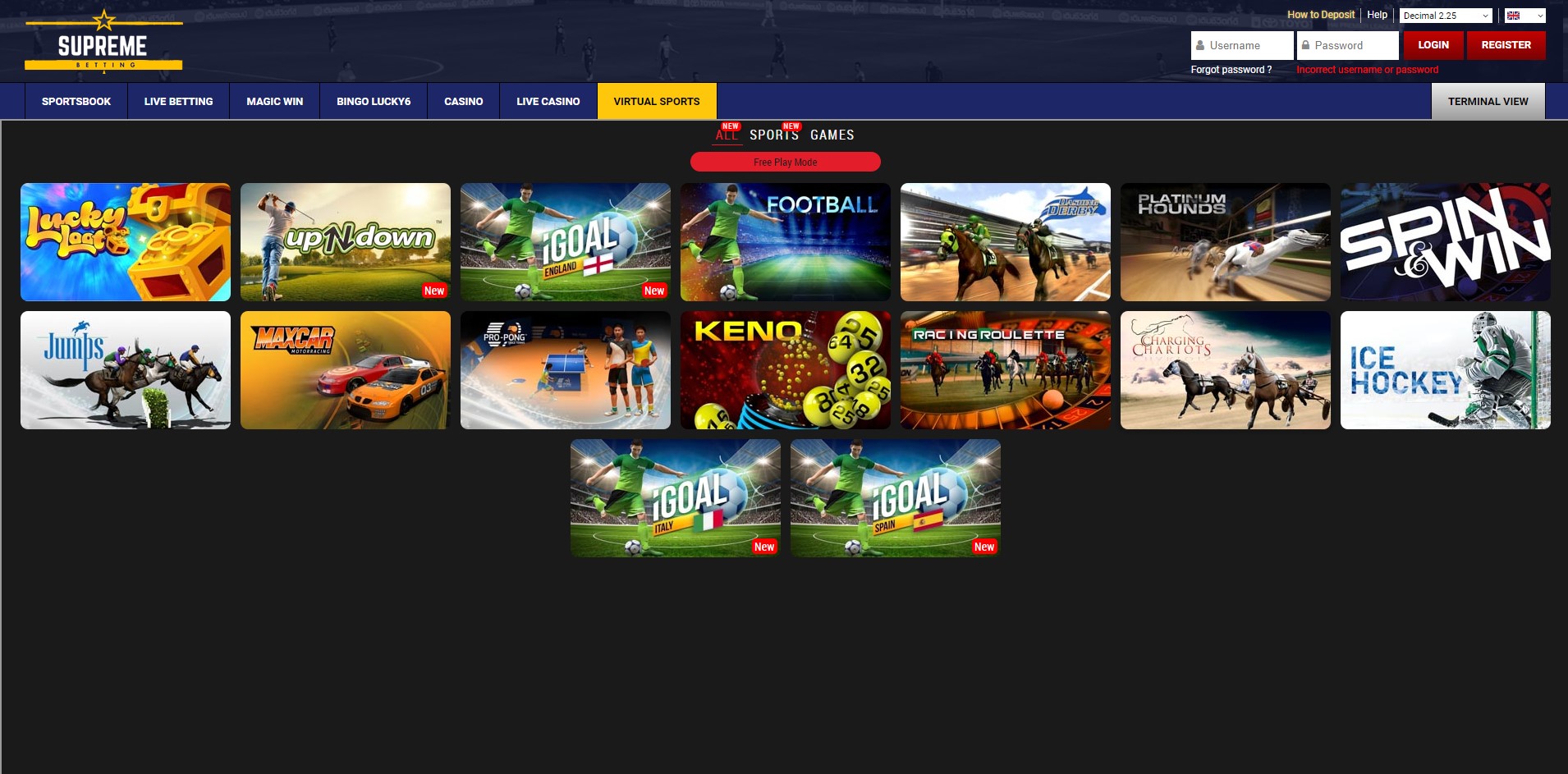This image showcases a diverse selection of games available on the Supreme Games and Gaming platform. Featured prominently on the game screen, players can access a variety of categories including sportsbook, live settings, magic wind, bingo luckies, casino, live casino, and virtual sports. The display highlights a series of specific games such as "Lucky Lou," "Up and Down" (a golf game), "Goal" (soccer), "Football" (soccer), "Horse Racing," "Platinum Hounds" (dog racing), "Spin and Win," "Ice Hockey," "Chariot Races," "Roulette," "Keno," and more. Additionally, the image depicts two individuals standing next to a small blue house with a truck driving away in the background. Following this, the game "Matt's Car" represents car racing, with another game featuring equestrian jumps where horses leap over obstacles. The last two games in the display are also soccer-themed. This snapshot provides an extensive overview of the gaming options available on this vibrant platform.